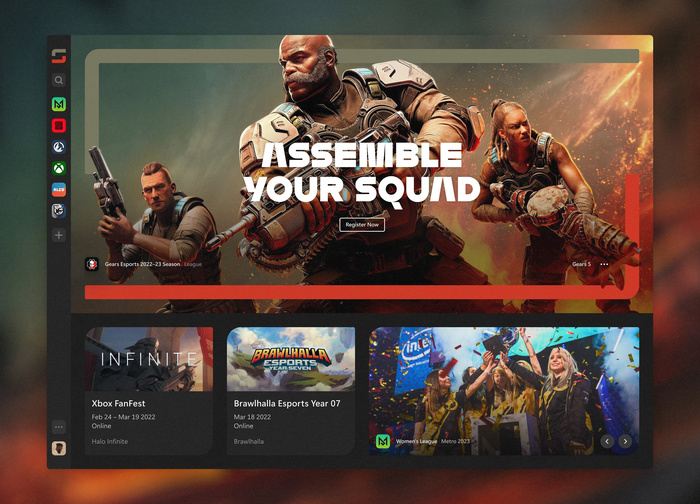The image titled "Assemble Your Squad" features a dynamic and intense scene, centered around a powerful, darker-complected man in the foreground. Clad in futuristic battle gear reminiscent of cartoon robotics, he stands as the focal point. His bald head is accentuated by a unique mustache and beard, intricately connected and flowing back over his ears, displaying a blend of black, brown, and gray hues.

Across his chest, the bold title "Assemble Your Squad" is emblazoned, drawing immediate attention. To his left stands a lighter-skinned man, similarly dressed in battle attire, though less heavily equipped. He wields a massive gun, adding to the sense of impending action. On the right, a figure who appears to be a woman with a darker complexion grips what resembles a rocket launcher, further heightening the image's combative energy.

Beneath the trio, an overlay of text reads "Infinite Brawlhalla Esports," accompanied by the Intel logo, indicating sponsorship. The celebratory atmosphere is enhanced by a cascade of confetti, suggesting a triumphant win and adding a vibrant, festive layer to the scene.